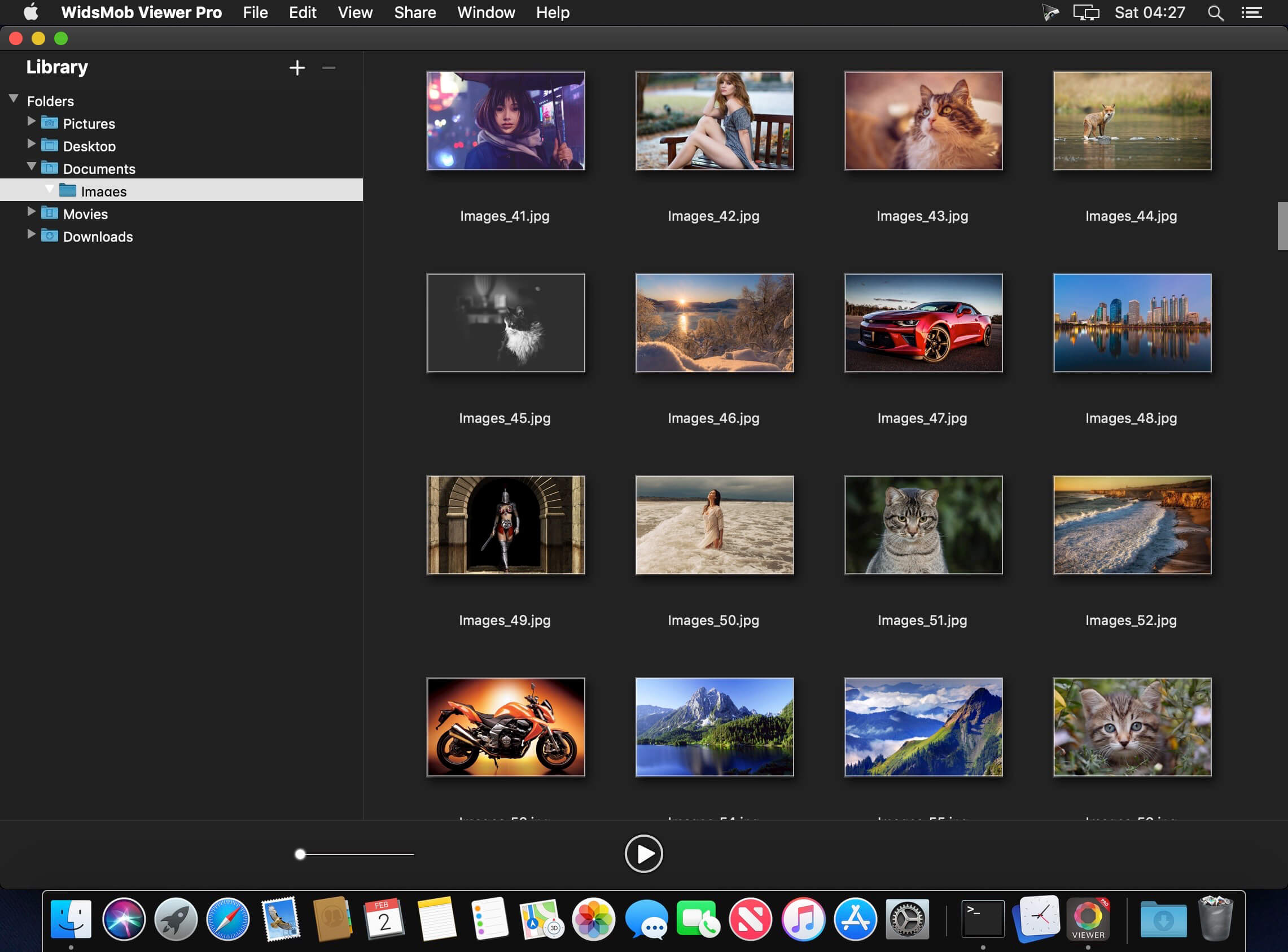This screenshot features the macOS operating system in dark mode, characterized by dark gray backgrounds and white text. The image displays the application "Widsmom Viewer Pro" open on the screen. At the top of the window, the menu bar options include File, Edit, View, Share, Window, and Help.

The taskbar at the top indicates the current time as Saturday at 4:27, though it does not specify whether it’s a.m. or p.m. 

The application window itself displays a hierarchical navigation menu on the left, with library categories such as Folders, Pictures, Desktop, Documents, Images, Movies, and Downloads. 

To the right, occupying the majority of the screen, is the main viewing area showing a grid of photo thumbnails. There are approximately four photos per row and four rows are visible, making a total of 16 thumbnails displayed. The filenames of these images follow a sequential numbering pattern starting at 41 and ending at 52 within this view. 

The images shown include various subjects such as a woman, a cat, and a car. Each thumbnail is a JPEG file, enhancing the application's utility as a comprehensive file viewer.